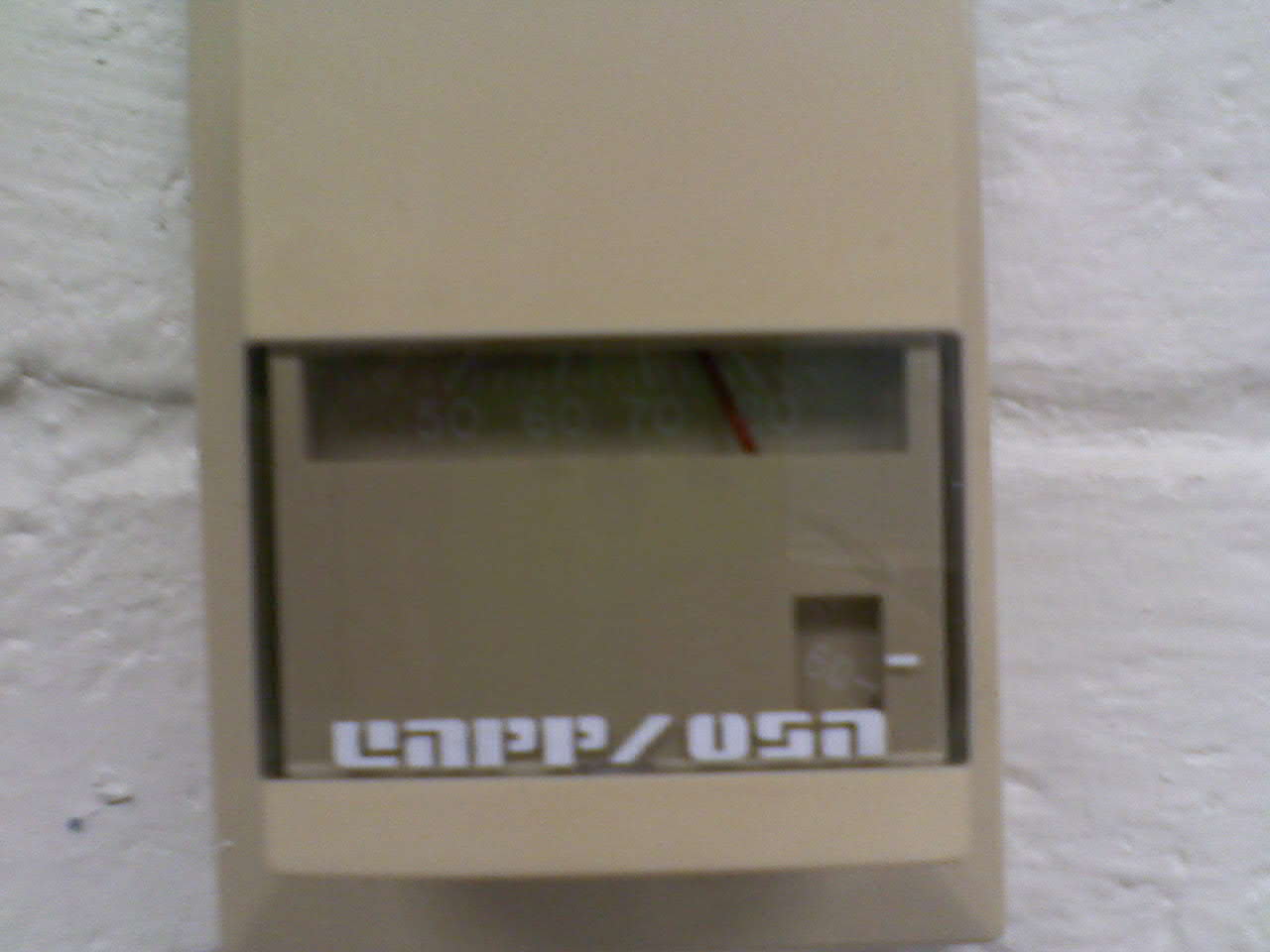The image captures an exposed, beige-colored thermostat with its cover removed, revealing its internal components. The face of the thermostat displays temperature markings in 10-degree increments, with a red needle positioned between 70 and 80 degrees, indicating a current temperature of approximately 75 degrees. A small, open box located in the lower right-hand corner of the display features some writing that is not clearly legible. Prominent, bold text at the bottom of the thermostat reads "CAPP/USA." The thermostat is mounted on a wall, which appears to be made of cinder blocks or bricks and painted entirely white.